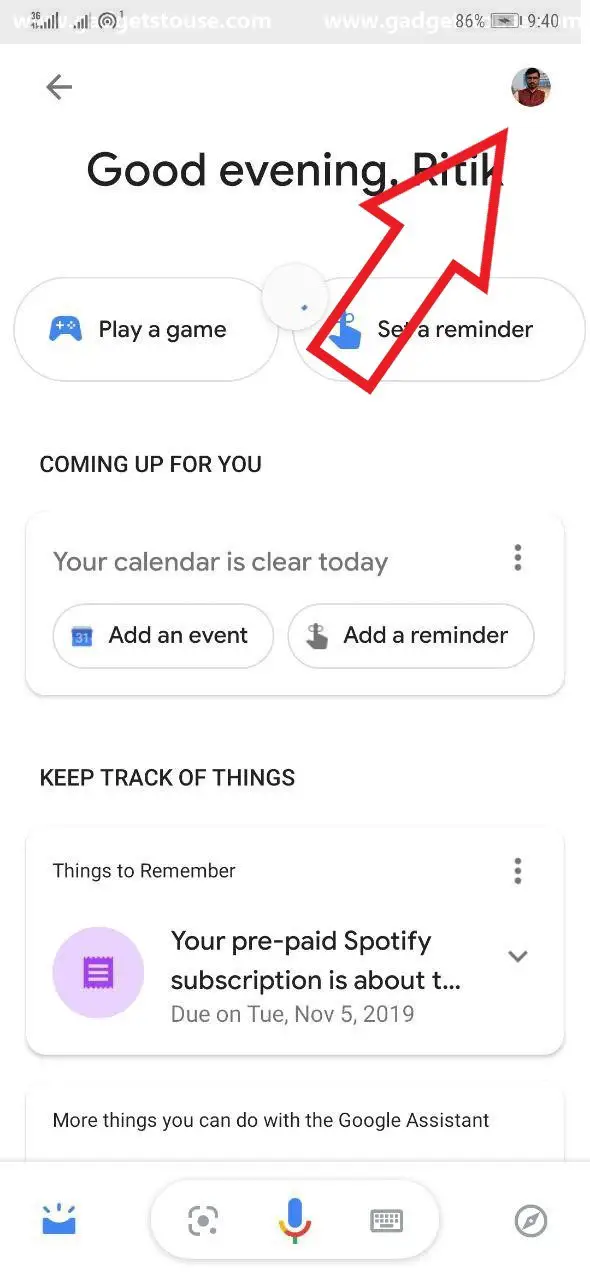Screenshot from a mobile app: 

At the very top, the mobile phone displays its connection to a network, 86% battery life, and the current time of 9:40 AM. On the app's interface, a profile icon featuring an image of a person is located in the top right-hand corner, highlighted by a prominent red arrow pointing towards it. Beneath this, the greeting "Good evening, Rich" is displayed in black text, although the last name, seemingly Ritik, is partially obscured by the red arrow.

Below the greeting, two pill-shaped buttons offer options to "Play a Game" or "Set a Reminder." Following these options, the section titled "Coming Up for You" appears. Within this section, it states, "Your calendar is clear today." Users are provided with two additional pill-shaped buttons to "Add an Event" or "Add a Reminder," accompanied by three ellipses in the top right-hand corner for more options.

Further down, there is a card labeled "Keep Track of Things - Things to Remember." It contains a truncated message "Your prepaid Spotify subscription is about to...," with a due date indicated as "Tuesday, November 5th, 2019."